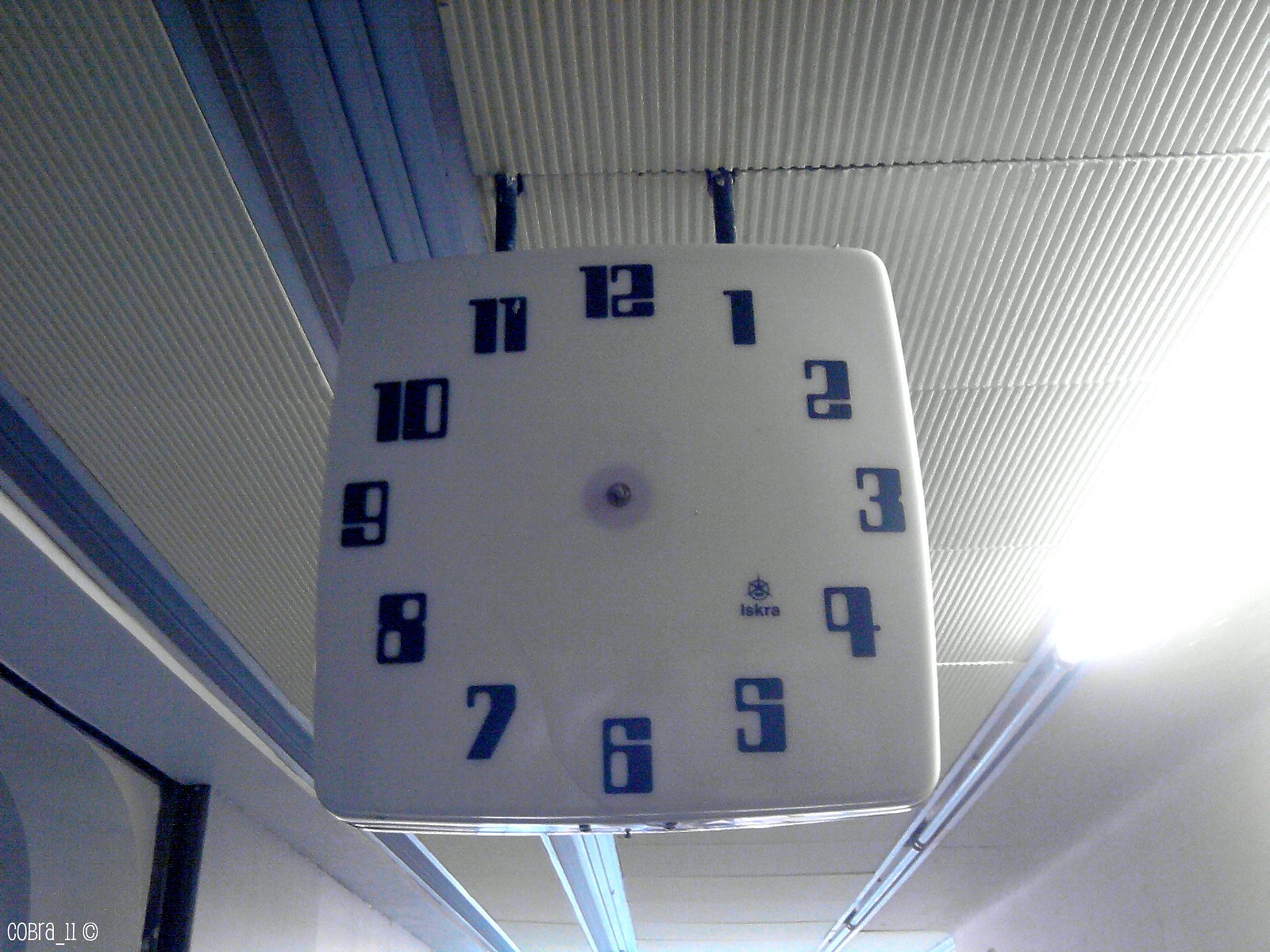The image depicts a large white square clock with blue numbers hanging from the ceiling in what appears to be a public transit area, possibly a subway or train station. The clock notably lacks hands, preventing any reading of the time. It is suspended by two blue clips attached to black rods against a white, corrugated roof with pronounced striations. A blue beam extends vertically down the left side of the ceiling. On the right side, a row of lights is visible with only the farthest one illuminated. The clock face features the inscription "LSKRA" between the 4 and 5 o'clock positions, suggesting a potential connection to a Greek location, further hinted at by the strong blue and white color scheme typical of Greek aesthetics. The overall scene is framed within architectural elements that contribute to a distinctly public and possibly international ambiance, reminiscent of a train station or airport.